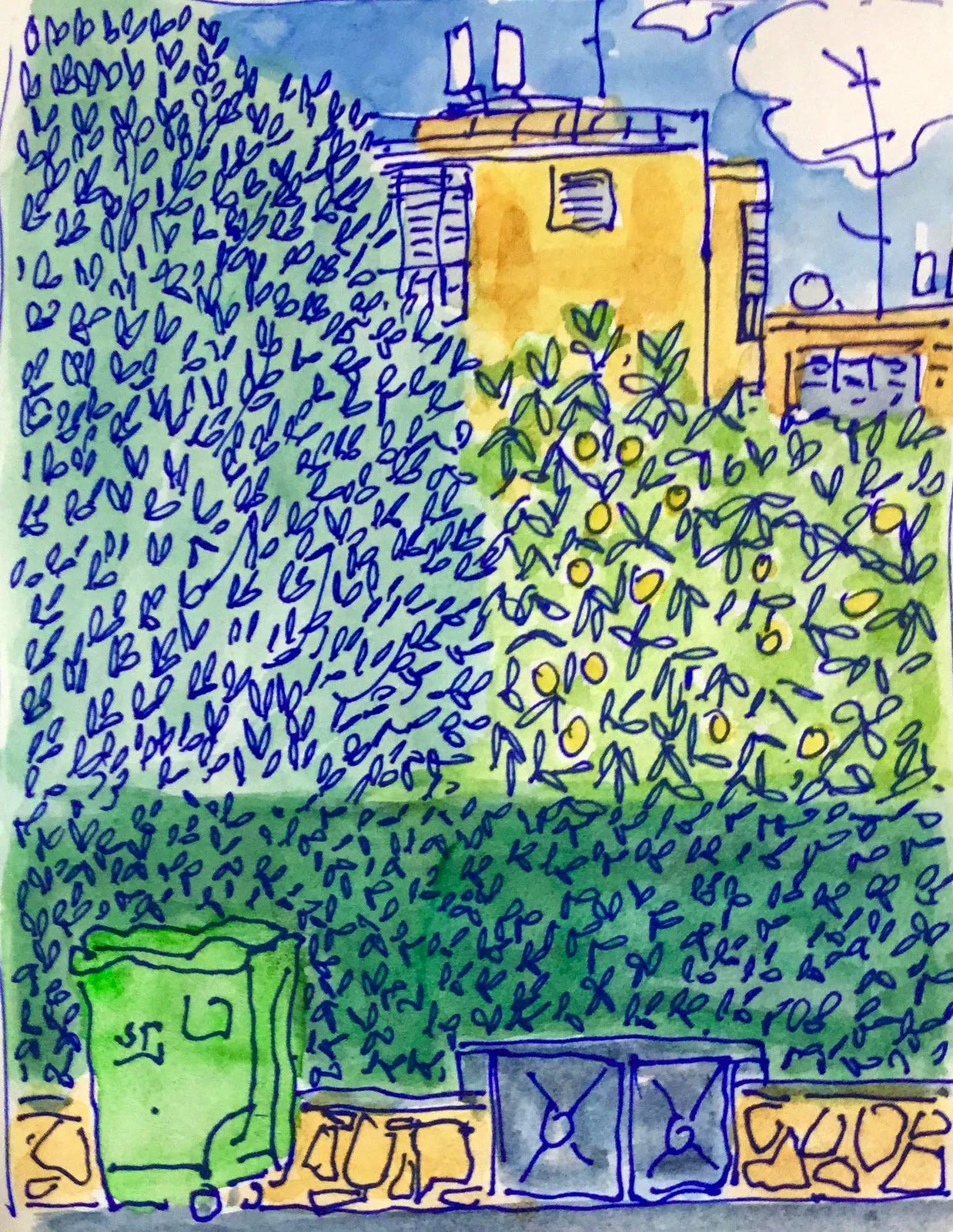The hand-drawn color illustration is presented in a portrait orientation and captures a snapshot of an urban environment. In the foreground, a blue recycling bin, cubic in shape, stands to the right, while a more upright green trash can with a lid and wheels is situated to the left. Both bins are positioned in front of a low, yellow stone wall. Adjacent to the wall, a dark green hedgerow details the scene with fine blue pen strokes. To the right of this hedgerow, a taller bushy plant, which resembles a lemon tree adorned with small yellow circles, adds to the depth. On the left, a much taller tree stands with lighter green foliage and intricate blue detailing for twigs stretching skyward.

In the background, the right side reveals a couple of buildings; one notably features white chimneys that evoke an industrial vibe, suggesting the presence of a polluting factory. This contrast with the recycling bins in the foreground might symbolize the juxtaposition between environmental pollution and efforts toward recycling. The buildings behind include windows shaded in blue and an orange roof, partly mingling with the blue sky and white clouds delineated by dark blue borders. The scene subtly conveys a commentary on environmental stewardship amidst urban surroundings.